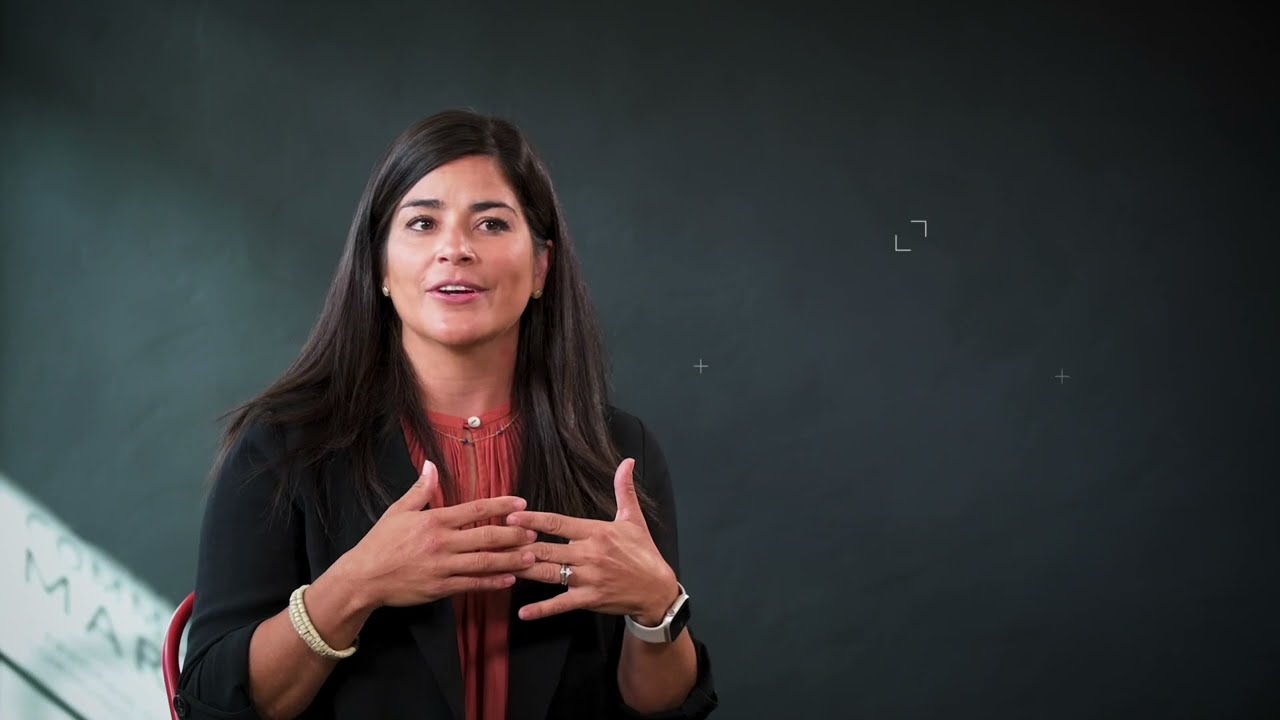The image features a young Caucasian woman, possibly in her late 20s to mid-30s, standing against a charcoal gray or dark chalkboard background that appears photoshopped. She is situated in the left third of the frame, with her left shoulder slightly angled towards the chalkboard. Her long, straight brown hair, parted on the side and tucked behind her ears, falls past her shoulders. Her eyebrows are dark and defined. She is wearing a reddish-orange blouse, buttoned at the collar, underneath a black or dark brown sweater. Around her neck, she has a small beaded necklace. Her attire also includes a gold bracelet on one wrist and a wristwatch on the opposite arm. A wedding ring adorns her left hand. The woman appears to be in conversation or talking, with her fingers interlocking in front of her chest. She is seated on what seems to be a metal red-backed chair. In the bottom left corner of the image, sunlight highlights partial text on the board that reads "COV" and "MAR."